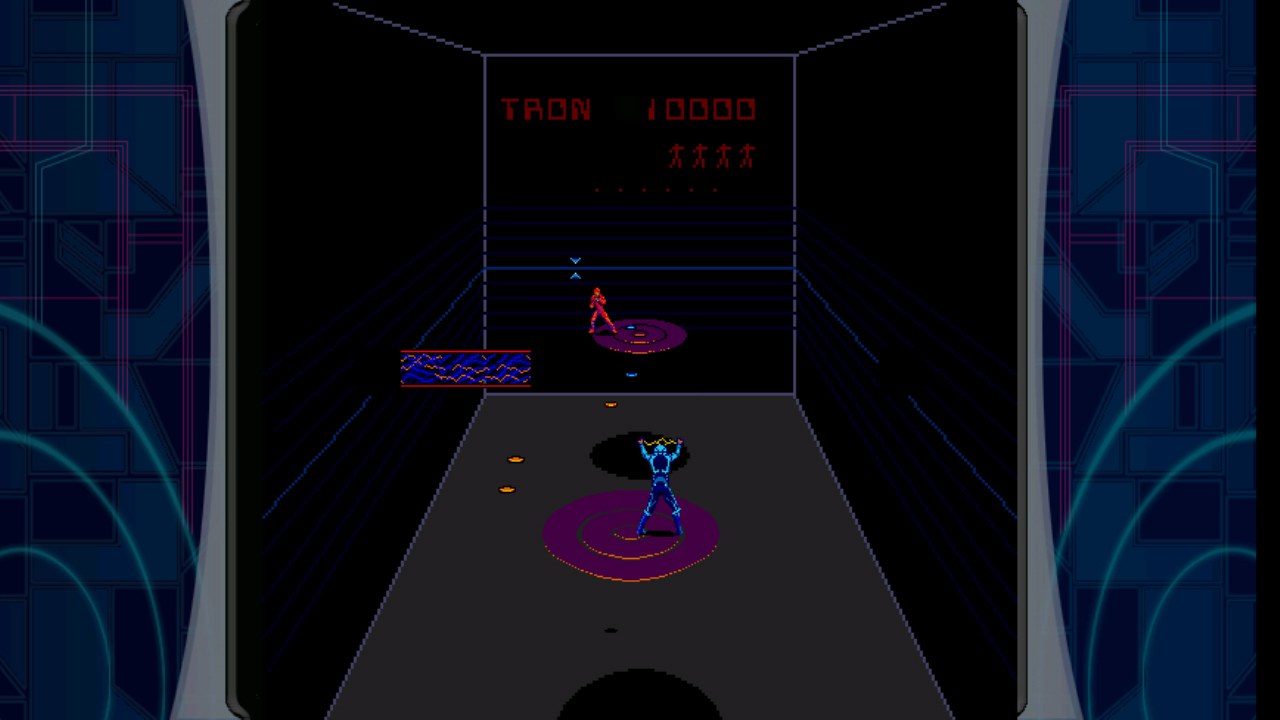A digital arcade cabinet displays a captivating scene from a Tron-themed game. The top of the cabinet proudly shows a "Tron 10,000 Score" label. The game appears to be set in a 3D space, designed for two players. At the top of the screen, a character on a red disc hovers ominously. The game arena is a vivid grid of intersecting lines: red lines stand out against a blue background, with additional orange lines adding complexity to the scene. Blue lines frame the left and right sides, interspersed with bits of pink, creating a visually engaging and dynamic playfield.